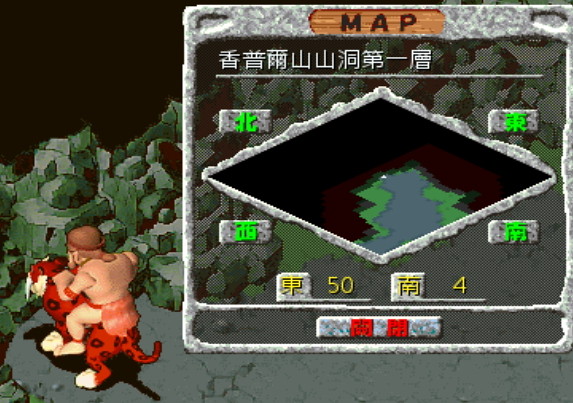This image is a screenshot of an older-style video game, seemingly in Japanese. Dominating the center to the far right is a prominent map screen, displayed as a sideways diamond outlined in white. The map features various colors such as black, red, green, and pale blue, with Japanese text indicating directions (north, east, south, and west). It also includes numbers like 50 and 4, and is set against a wood-colored background with green rock-like structures to the left of it. In the bottom left corner of the image, a muscular, tribal-like man wearing a caveman-esque loincloth and a bandana can be seen. He is riding a red cheetah with black spots, both facing away from the viewer. The little white dot on the map likely represents the player's current location in the game world.